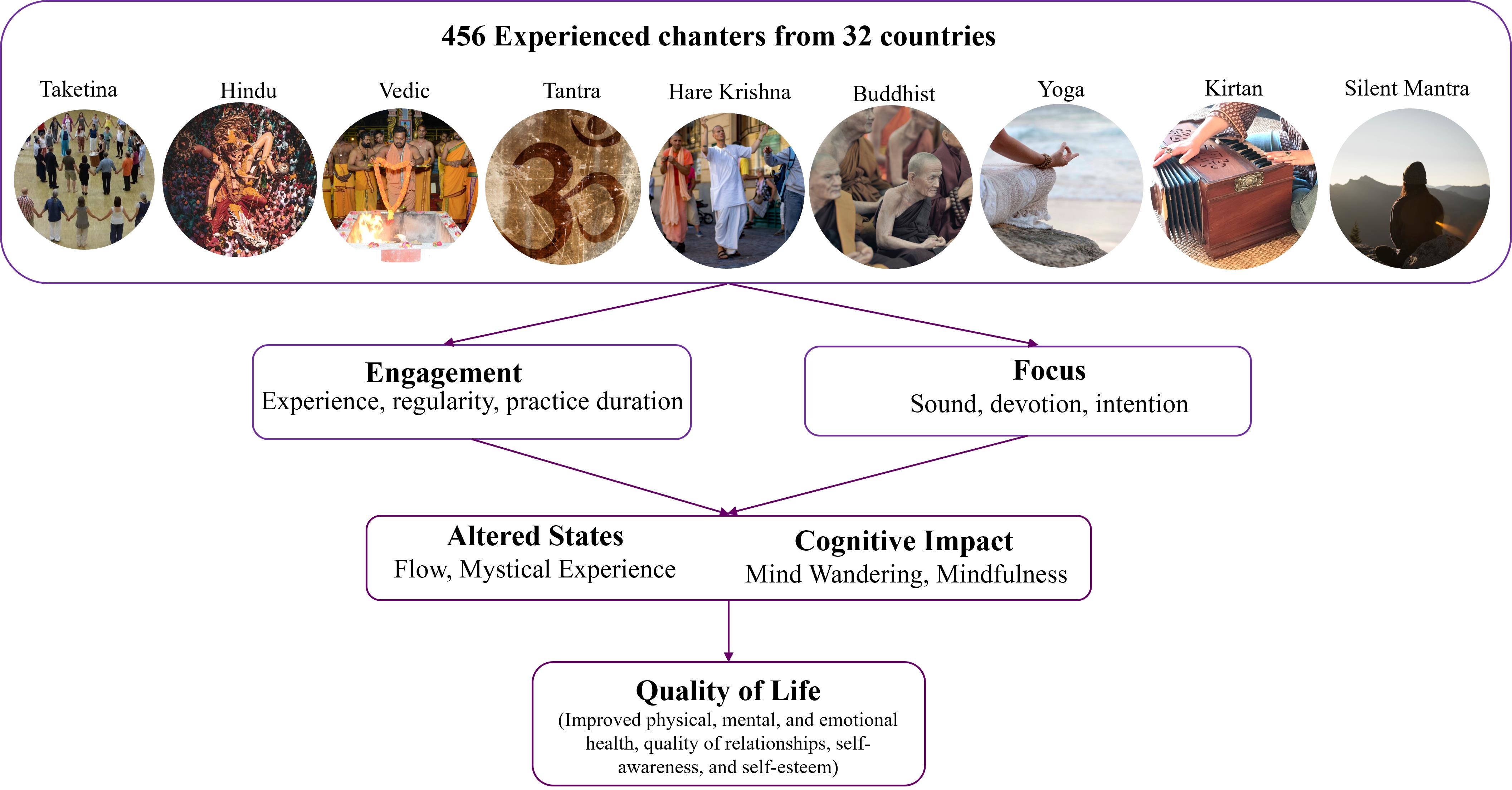The image is a detailed PowerPoint slide depicting an elaborate organizational flowchart. At the top is a large rounded rectangle, featuring the bold text "456 experienced chanters from 32 countries." Inside this rectangle are nine circles, each containing images and a label corresponding to different chanting traditions. From left to right, the circles are labeled: Taketina, Hindu, Vedic, Tantra, Hare Krishna, Buddhist, Yoga, Kirtan, and Silent Mantra.

Below this top rectangle, two purple arrows point downwards to two smaller rounded rectangles. The left rectangle is titled "Engagement" in bold and includes subtext: experience, regularity, practice, duration. The right rectangle is labeled "Focus" in bold, with subtext: sound, devotion, intention.

These two rectangles converge into a larger, unified rectangle. On the left side of this rectangle, in bold text, it reads "Altered States," with subtext: flow, mystical experience. On the right side, it is labeled "Cognitive Impact," with subtext: mind wandering, mindfulness.

A final arrow extends downward from this large rectangle leading to the bottom rectangle, labeled "Quality of Life" in bold. Underneath, in smaller text, it reads: improved physical, mental, and emotional health, quality of relationships, self-awareness, and self-esteem. This comprehensive chart integrates various aspects of chanting traditions and their impact on practitioners' lives.